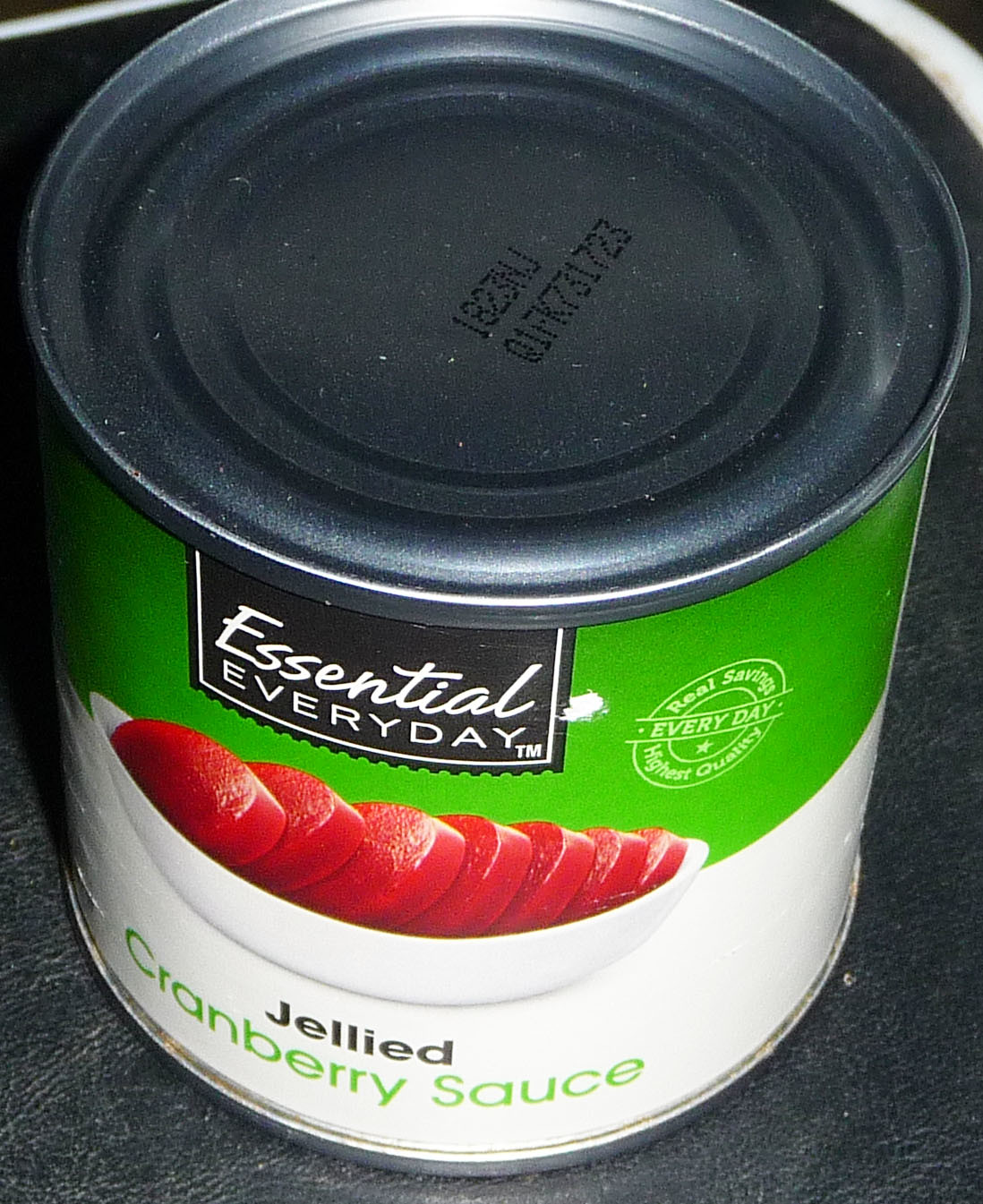The image showcases a product with a label depicting various elements. At the center of the label, there is a brown background that is intended to represent black leather. At the very top of the label, there is a silver section. The top of the product label features a green sticker with the text "Real Savings, Everything in Higher Quality." Below this green sticker, there is a black label that prominently displays "Essential Everyday." The lower part of the label shows a white bowl containing multiple red slices, which appear to be fruit slices. At the bottom of the label, the word "Jelly" is visible, with "Cranberry Sauce" written in green text above it. Additionally, there is a noticeable accumulation of dust on the image. At the very bottom edge of the product label, there is a silver lip.